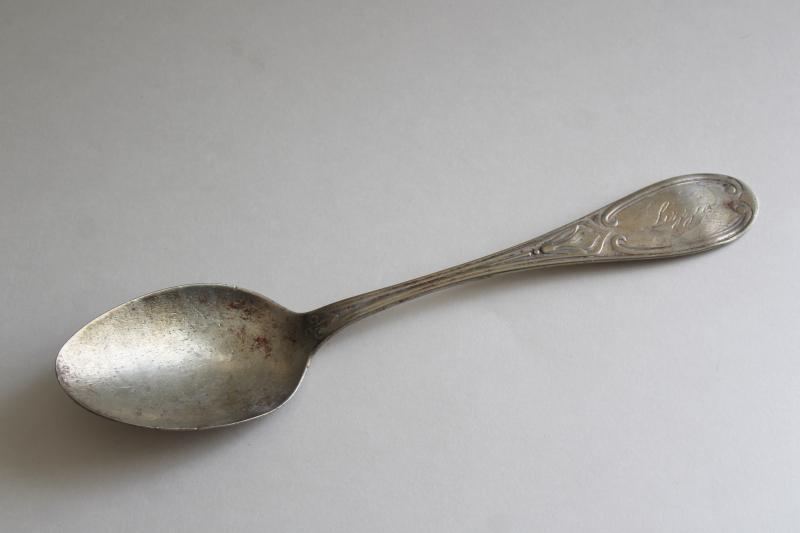This photograph showcases a single, antique spoon, made of tarnished and slightly rusty silver, centered against a grayish-white background. The spoon is oriented with the bowl on the left and the handle on the right. It features a subtle design pattern on the handle and carries a barely legible cursive inscription, possibly reading "Lizzie." Notably, there is a red rust spot at the tip of the handle and additional tarnishing within the bowl area, hinting at its age and extensive use. The background appears to be a whitish surface, such as paper or a table, which further highlights the spoon as a historical artifact.